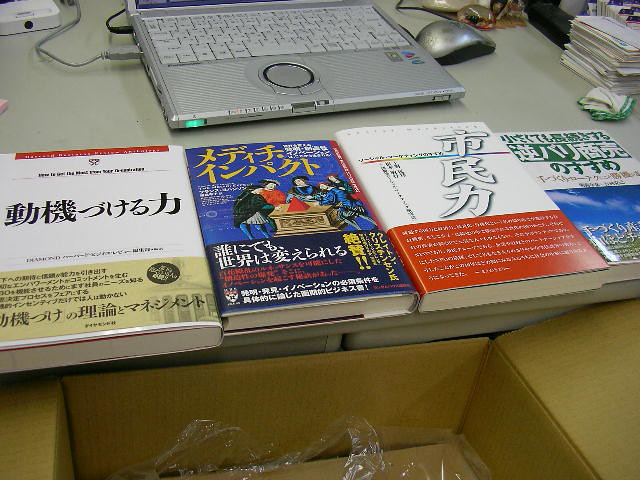The photograph captures a detailed scene of a green-tinted work or study desk, viewed from the perspective of someone sitting behind it. Central to the image is an opened cardboard box placed just in front of the desk, containing torn plastic wrappings. 

On the desk, four books with non-English inscriptions, likely Japanese or Chinese, are arranged from left to right at the edge. The first book on the left is mostly white with a yellow block, the second book features a blue cover with an old-fashioned illustration of people, the third book is primarily white with a red rectangle at the bottom, and the fourth book transitions from white at the top to blue at the bottom.

Behind the row of books sits an old, bulky silver laptop, reminiscent of early 1990s models, with a rounded mouse pad area. To the right of the laptop is a sleek gray mouse with a black base. The desk also holds various papers and possibly other small items like a paperweight, contributing to the perceived function of the area as a working or studying space.